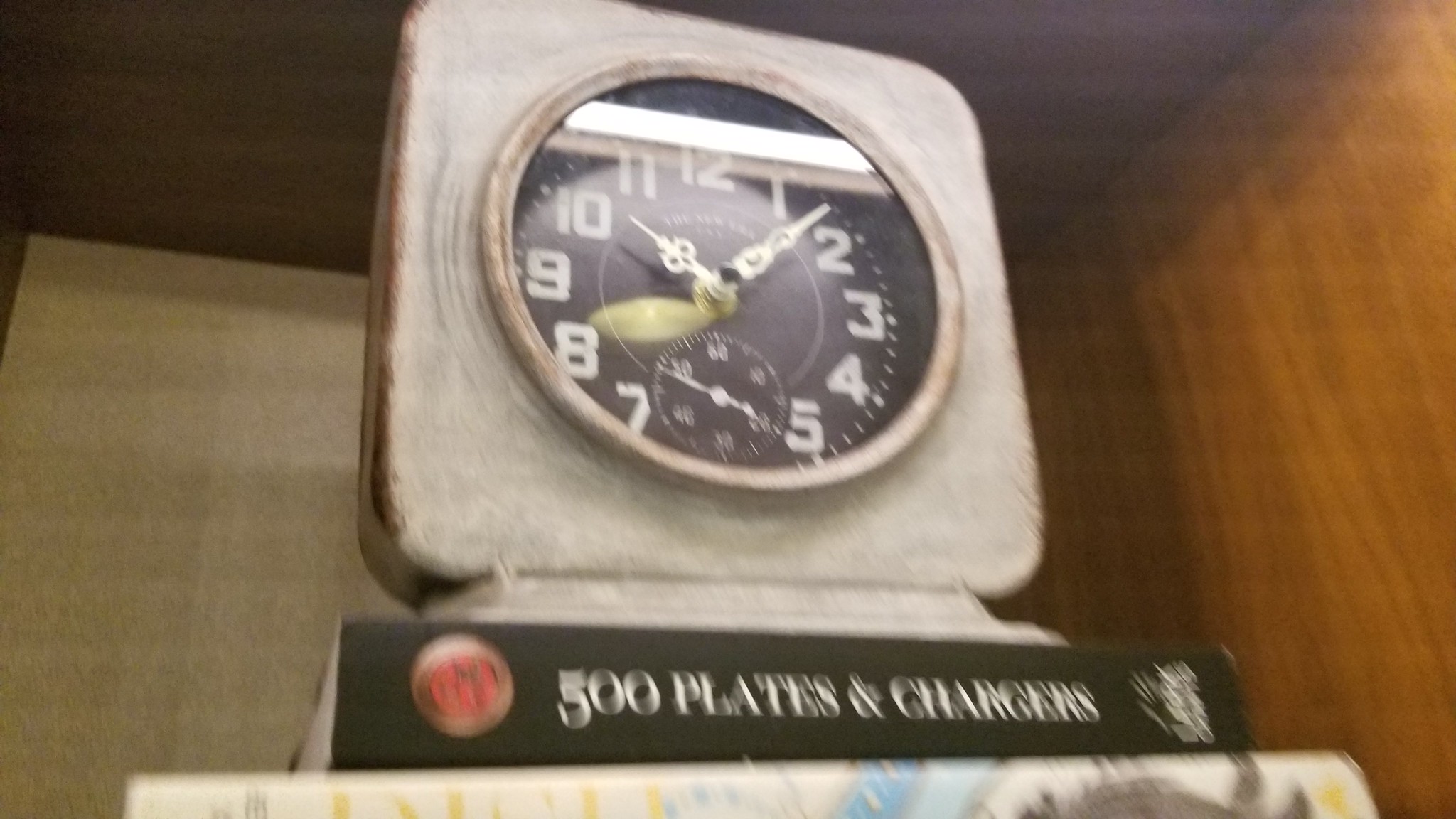In this close-up, slightly blurry photograph, a square clock rests atop a couple of stacked books. The background features a distinctive blend of textures, with a brown wood grain wall on the right side and a cream-colored wall behind. The clock itself is unique, set on a sturdy stone base, and showcases a round clock face encircled by a sleek metal border. The clock face is black, displaying white numerals and elegant, gold-engraved hands that indicate the time. Beneath the main hands, a smaller subdial features an additional hand for tracking seconds. A fluorescent ceiling light is reflected on the clock's glass face, adding an extra gleam to the scene.